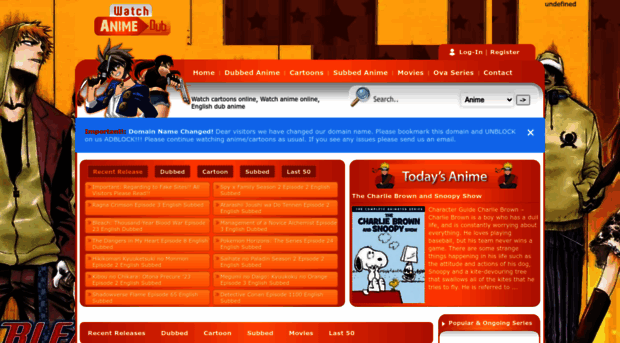This image is a blurred screenshot of a webpage likely dedicated to purchasing anime content. The background features an anime-style animation with vibrant colors and intricate details. A prominent banner in the center of the image states "Watch Anime." On the left side of the banner is an illustration of a man in a hooded jacket, accompanied by several other anime characters, adding a dynamic and engaging visual appeal.

At the top of the page, there is a navigation menu with options listed from left to right: Home, Dubbed Anime, Cartoons, Subbed Anime, Movies, OVA Series, and Contact. In the top right corner, there are links for "Log In" and "Register," providing easy access for users to manage their accounts.

A blue bar spans across the top of the page, featuring some white text which is unfortunately unreadable due to its small size and blurry appearance. Below this bar, the layout is divided into two columns, both with an orange background and white text that is also too small and blurry to decipher clearly. The right column contains an image of Snoopy from the Peanuts series, accompanied by partially readable text stating "The Charlie Brown and Snoopy," followed by an indecipherable word.

Overall, this screenshot captures the essence of an anime-focused website with a detailed and visually appealing layout, hampered only by the lack of clarity in the text.